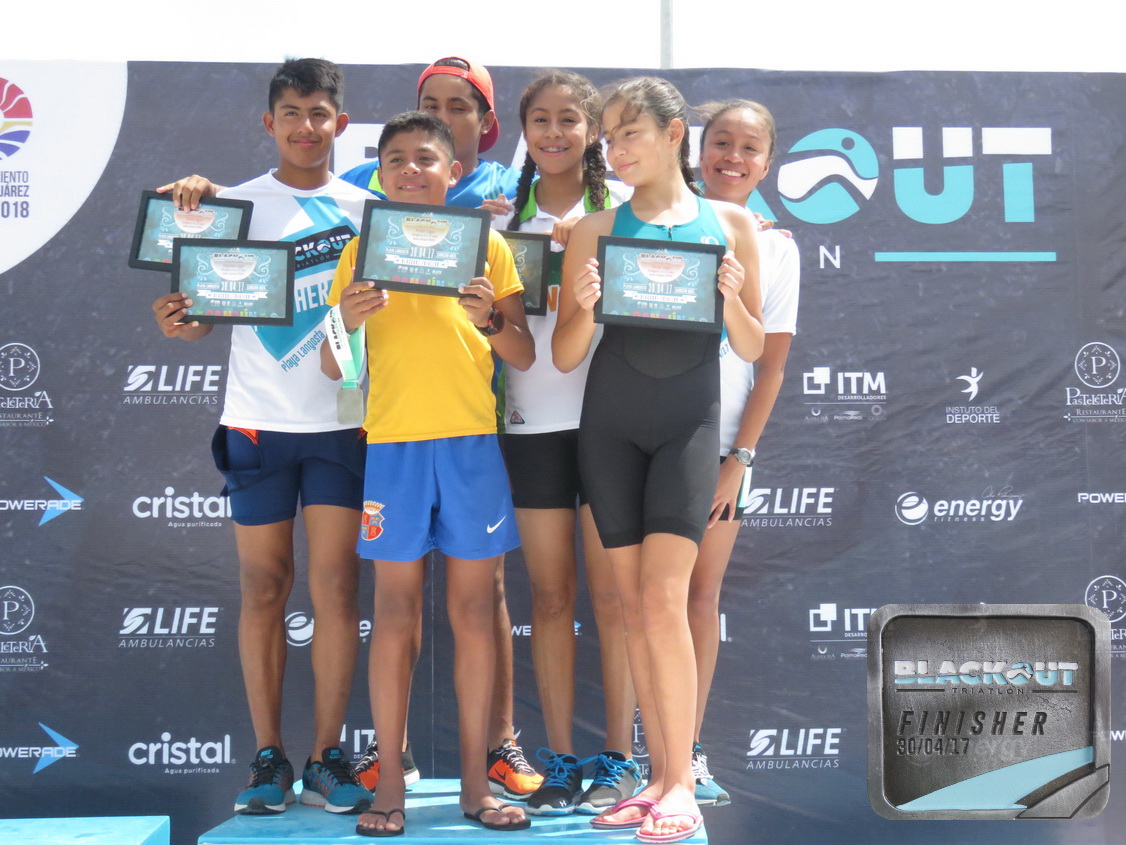A group of young children, likely around 9 or 10 years old, are gathered on a light blue platform in front of a step-and-repeat backdrop filled with various advertisements and logos, including "Energy," "Life Ambulances," and "Crystal." The backdrop also features a circle with blue, white, and black colors alongside the letters UNT in blue and white, as well as a gray square at the bottom right that states "Blackout Triathlon Finisher 30-04-17."

The children are holding a black-framed picture, showing an image of a trophy against a blue background, instead of an actual trophy. From left to right:

- The farthest left is a boy with short black hair, smiling, wearing a white shirt, blue shorts, and blue shoes.
- In the forefront stands the smallest child, also with short black hair, clad in a yellow shirt, blue shorts, and sandals.
- Behind the smallest child is a person with an orange cap worn backwards, eyes closed.
- Next to the person with the cap is a smiling girl with braids over her shoulders, dressed in a white shirt with a green collar and black shorts.
- In front of this braided girl is another girl whose head is turned to the left, wearing a black and turquoise swimsuit resembling a unitard and sandals.
- On the far right, another smiling girl leans her head slightly towards the left. She wears a white shirt and has a watch on her wrist.

Most of the children appear to be in swimming attire, with a mix of sneakers and sandals on their feet, highlighting a blend of casual and athletic dress.